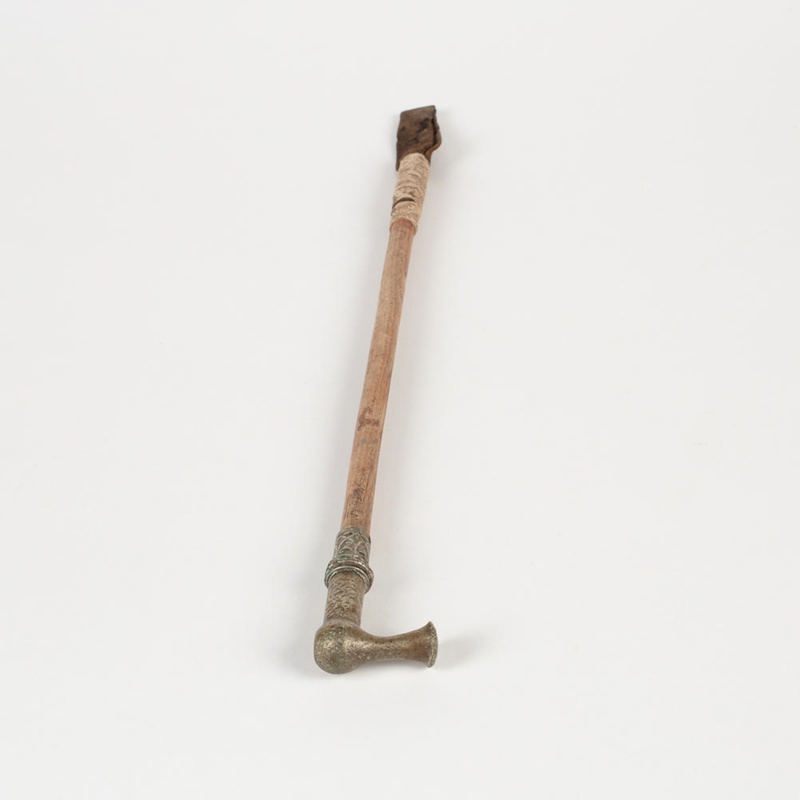The image shows what seems to be an antique wooden cane, laying on its side against a plain white background. The handle, which resembles an L-shaped doorknob or a bicycle horn, is crafted from a hard, dark material that may be iron or a dull metallic finish. This handle smoothly transitions into the wooden shaft, which is the longest part of the cane and features intricate, finely carved details. The wood appears aged with muted, neutral tones. A piece of string or thin rope is wrapped around the lower part of the cane, leading to a thicker, darker brown section at the end, which looks either burnt or intentionally darkened for visual contrast and added support. The overall color scheme is subdued, consisting of grays, muted browns, and natural wood hues, with no bright or vivid colors.